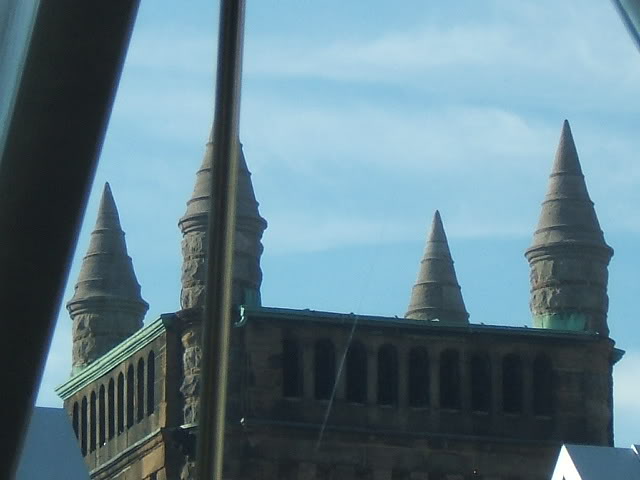The image depicts a tall, weathered stone tower set against a light blue sky dotted with puffy white clouds. The tower, which appears old and constructed from dark gray stone, features four cylindrical turrets with pointed, cone-like tops at each corner, seamlessly matching the color of the main structure. Near the top of the tower, there are tall, arched windows with flat bottoms that curve into graceful arches. The building shows signs of age, with some sections exhibiting green discoloration from oxidized copper. The scene is partially obstructed by metal bars, likely part of a bridge or a nearby structure, positioned diagonally from the bottom left corner to the top left, and another running upright on the right side of the image. Additionally, the peak of another building, triangular and white-gray, is visible in the bottom right corner.